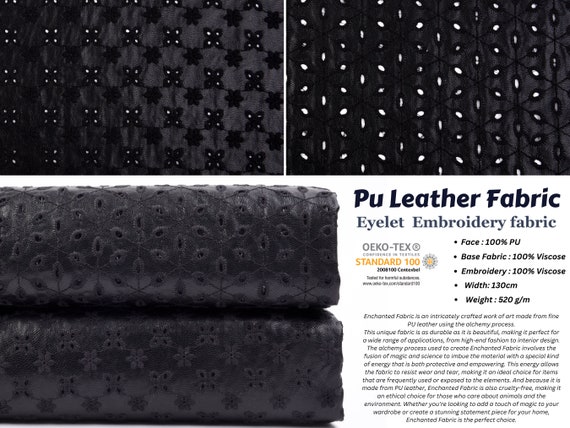The image showcases various types of black fabrics, labeled as PU leather fabric and eyelet embroidery fabric. These fabrics are characterized by detailed perforations, creating intricate patterns. One fabric displays a repeating grid pattern of star shapes alternating with X shapes, while the other features a hexagonal snowflake design with six perforated holes. Both fabrics are neatly folded into stacks. The detailed description provided specifies that the face material is 100% PU, the base fabric is 100% viscose, and the embroidery is 100% viscose, with dimensions of 130 centimeters in width and a weight of 520 grams per meter squared. Additional fine print includes further descriptions of the fabric's manufacturing process, all in black lettering.